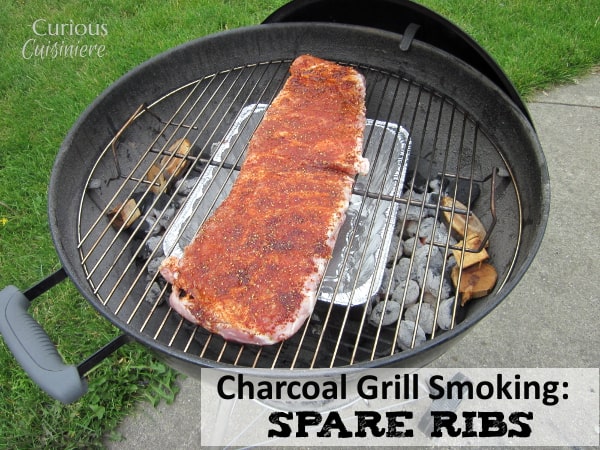This close-up image showcases an old-timey, circular, black barbecue grill, reminiscent of a classic Weber design. Positioned on a split surface, with neatly trimmed green grass on the top-left and a gray cement sidewalk on the bottom-right, the grill dominates the center. The grill's black lid is hooked to its side, while charcoals are visible at the bottom, preparing to cook a large, highly seasoned, nearly red rack of spare ribs atop the grill plate. Beneath the grill plate, an aluminum container, possibly catching juices and providing moisture, awaits the cooking process. The front of the grill features a gray handle and a small rectangular label reading "charcoal grill smoking: spare ribs," confirming the culinary treat. Additional text, "Curious Cuisiner," hints at the playful and experimental nature of the chef behind the grill.